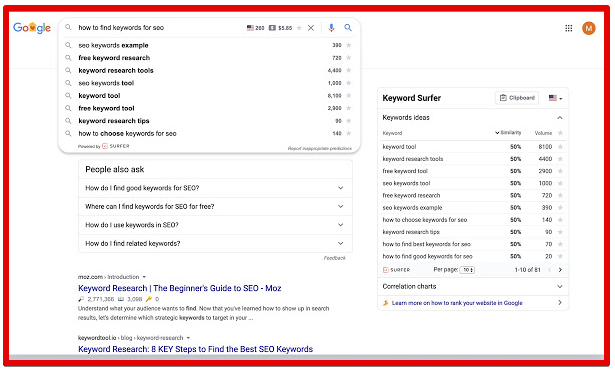The image displays a website featuring an interface with a prominent red border around its edges and a white background. At the top of the page, there is the "Google" logo, adjacent to a search bar with the query, "how to find keywords for SEO" typed in. 

Below the search bar, a list of keywords and phrases is presented, including:
- Free keyword research example
- Keyword research tools
- SEO keywords tool
- Free keyword tool
- Keyword research tips
- How to use keywords for SEO

Near the top right corner, an American flag icon, a microphone icon, and a magnifying glass icon are visible.

Further down the page, there's a section titled "People also ask," listing frequently asked questions related to keyword research, each with a dropdown menu. The questions include:
- How do I find good keywords for SEO?
- Where can I find keywords for SEO for free?
- How do I use keywords for SEO?
- How do I find related keywords?

At the bottom of the image, there is a feedback link labeled "Send feedback" next to text stating, "Keyword research: A guide to SEO." Below that, in blue text, it reads, "Key steps to find the best SEO keywords."